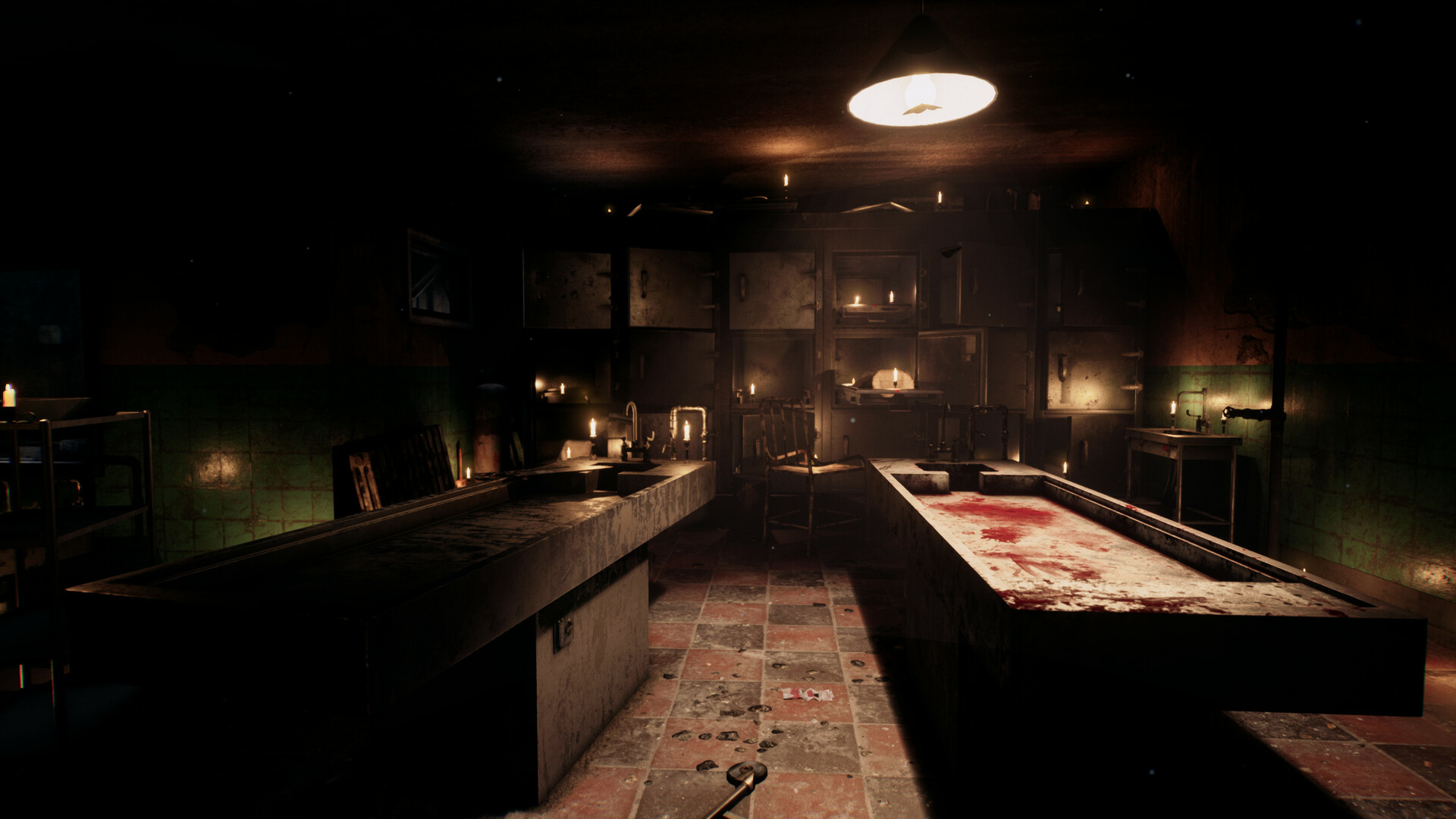In the image, an eerie, dark room is illuminated primarily by a single ceiling light with a dome shape, casting a stark light onto two central tables. The tables, reminiscent of air hockey tables in size and shape, appear to be constructed from cement or a similarly hard material. The table on the right is notably stained with what looks like blood, suggesting it may have been used for grim purposes such as torture, dismemberment, or autopsies. This table also features a rectangular cutout at one end. The table on the left remains shrouded in darkness, its use and condition obscured by the low light. The room itself is devoid of natural light and contributes to the unsettling atmosphere with its checkered floor pattern of red and brown squares, which are dirtied and scratched. In the dimly lit background, lit candles are scattered across shelves and open cabinets, adding to the macabre feel of the space. Other visible elements include desks, chairs, and a sink area, reinforcing the notion that this forsaken room could serve as a disturbing scene out of a horror or crime drama.